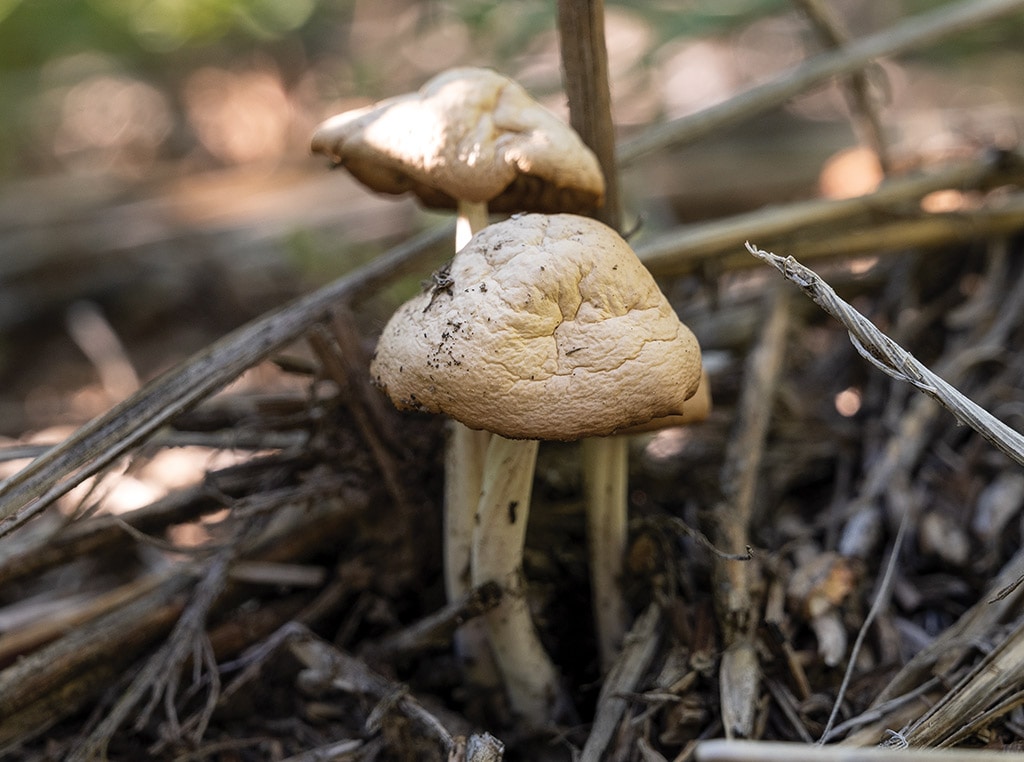This full-color photograph captures a close-up view of two white, semi-dried mushrooms growing outdoors in the daylight. Taken from ground level, the square image centers on the two mushrooms amidst a backdrop of decaying twigs, dead grass, and foliage. The caps of the mushrooms are cream-colored, transitioning to tan and black along the edges, and display visible cracks and dirt. The shorter mushroom is positioned in front of a taller one, both exhibiting cream-colored stems. Sunlight dapples the scene, illuminating one mushroom while leaving the other in shadow. The natural setting features a blurred background with hints of brown and green, enhancing the earthy, organic feel of the image.